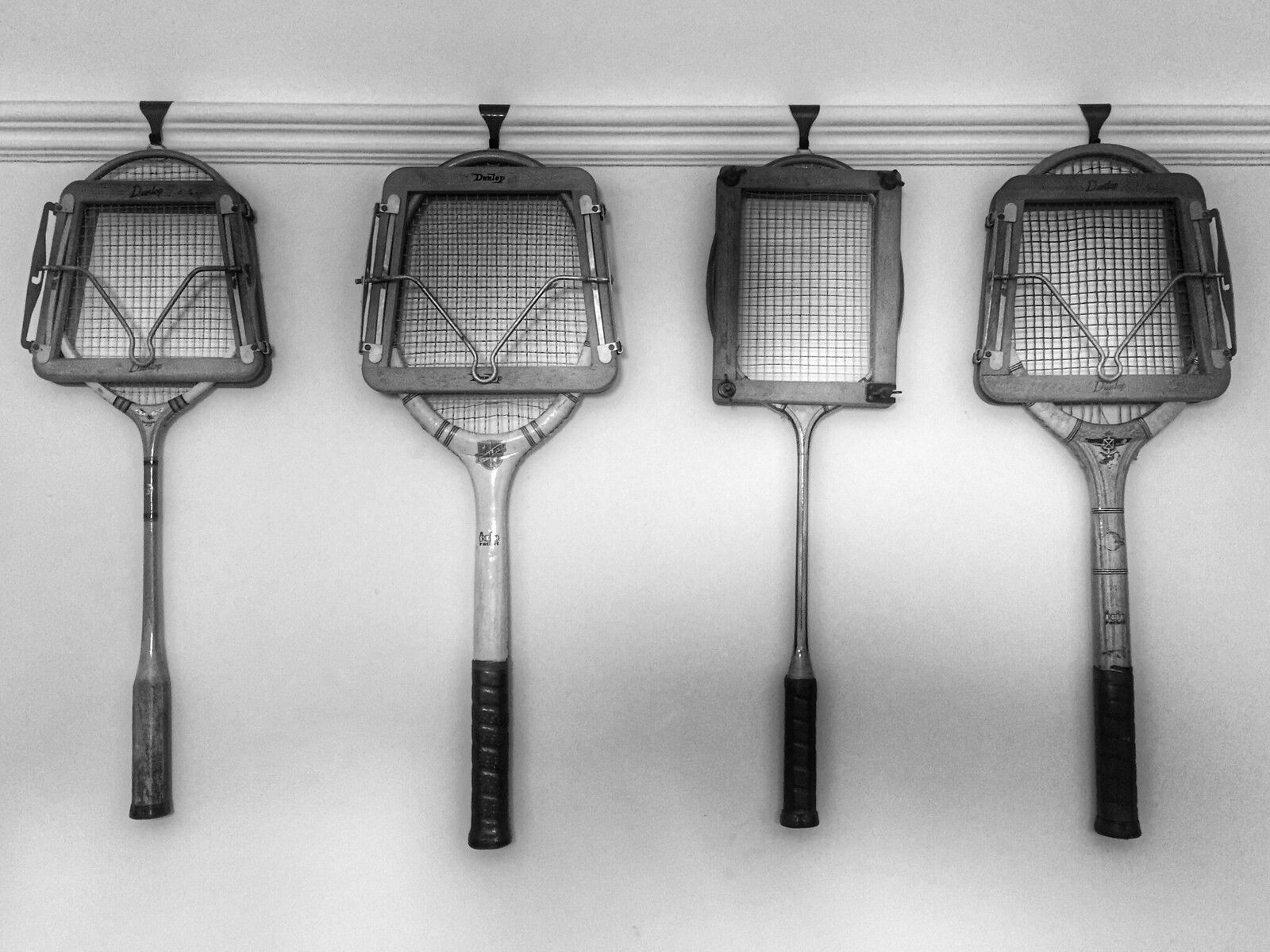The photo depicts four vintage tennis rackets hanging on a well-lit, white wall, each encased in unique wooden frames that have an irregular, rectangular shape. The rackets themselves are visibly old, indicated by their wooden handles, which feature black tips and black tape-like riveting. Three of the rackets have larger, oval-shaped heads, while one has a noticeably smaller head and thinner handle. Attached to each racket, a black mesh net with a square grid pattern fills the oval heads. The wall includes hooks on rounded edges to support the display of these distinctive pieces, making the rackets look like they are framed pieces of art. Logos or decals can be seen near the top of the handles, adding a touch of detail to these antique sporting items.